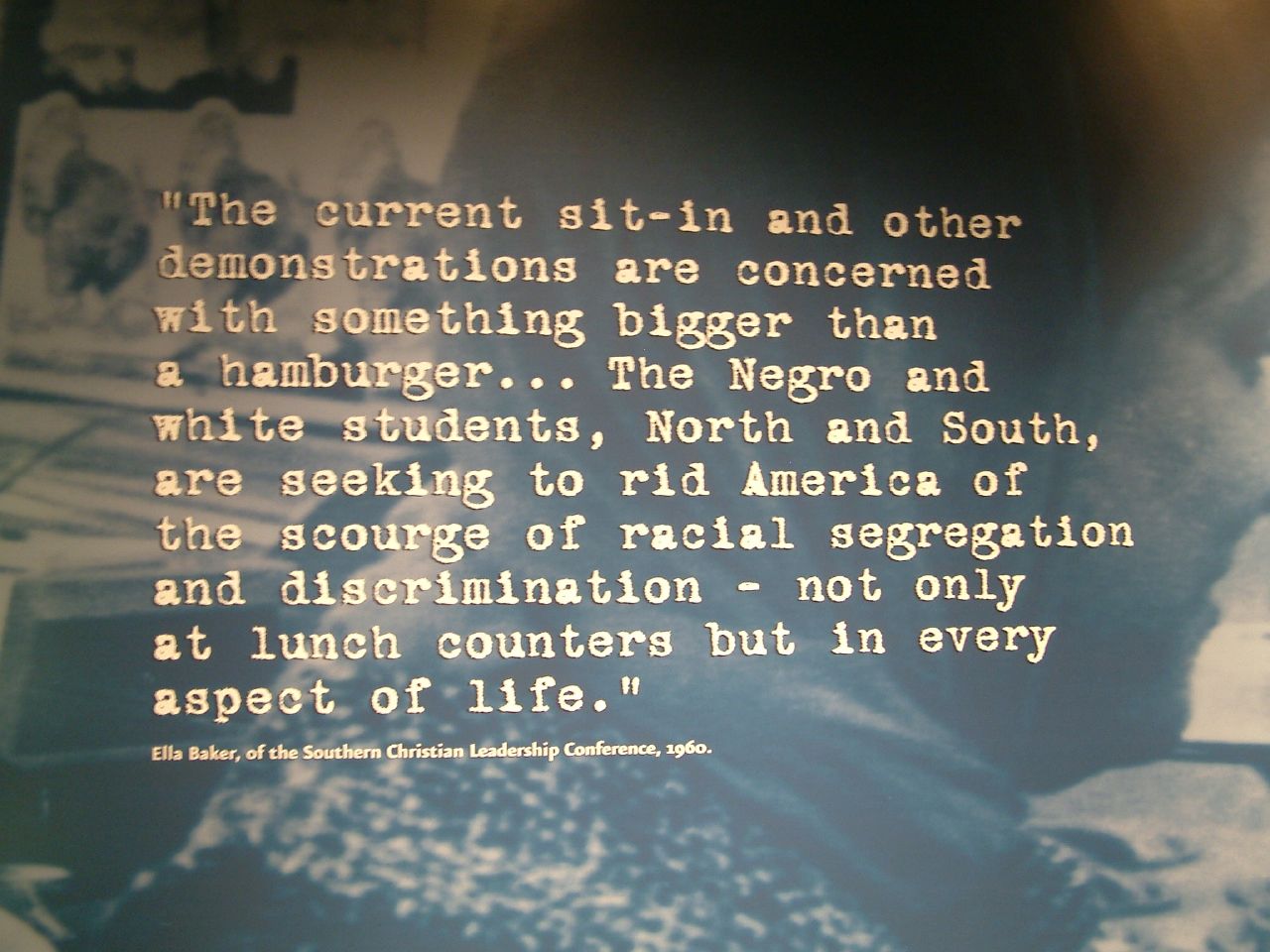The image features a powerful motivational message set against a faded black-and-white photograph of a woman crying, potentially Ella Baker. The focal point of the image is a quote by Ella Baker from the Southern Christian Leadership Conference in 1960. The quote reads, "The current sit-in and other demonstrations are concerned with something bigger than a hamburger. The Negro and white students, North and South, are seeking to rid America of the scourge of racial segregation and discrimination not only at lunch counters but in every aspect of life." The text is prominently positioned in the center, using white font on a black background, drawing attention to the significance of the Civil Rights Movement.